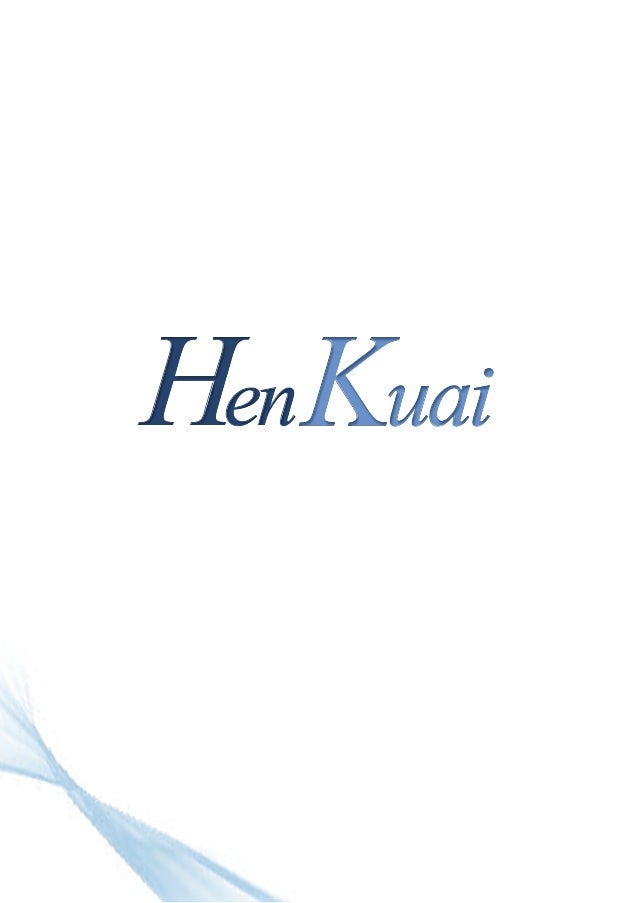The image is a poster set against an all-white background featuring text and a stylized design. Centered in the middle of the poster is the text "HEN KWAI." The word "HEN" is written in dark blue or black letters with a capital 'H' followed by lowercase 'e' and 'n'. The word "KWAI" follows without any space, with a capital 'K' and lowercase 'uai' in a greyish or sky blue font. The text appears italicized. In the bottom left corner of the poster, there is a stylized ribbon-like design resembling twisted gauze or a flowing stream of water. This design starts more condensed in the upper left and spreads out as it moves downward to the bottom left, with the ends being darker blue than the more transparent middle section.